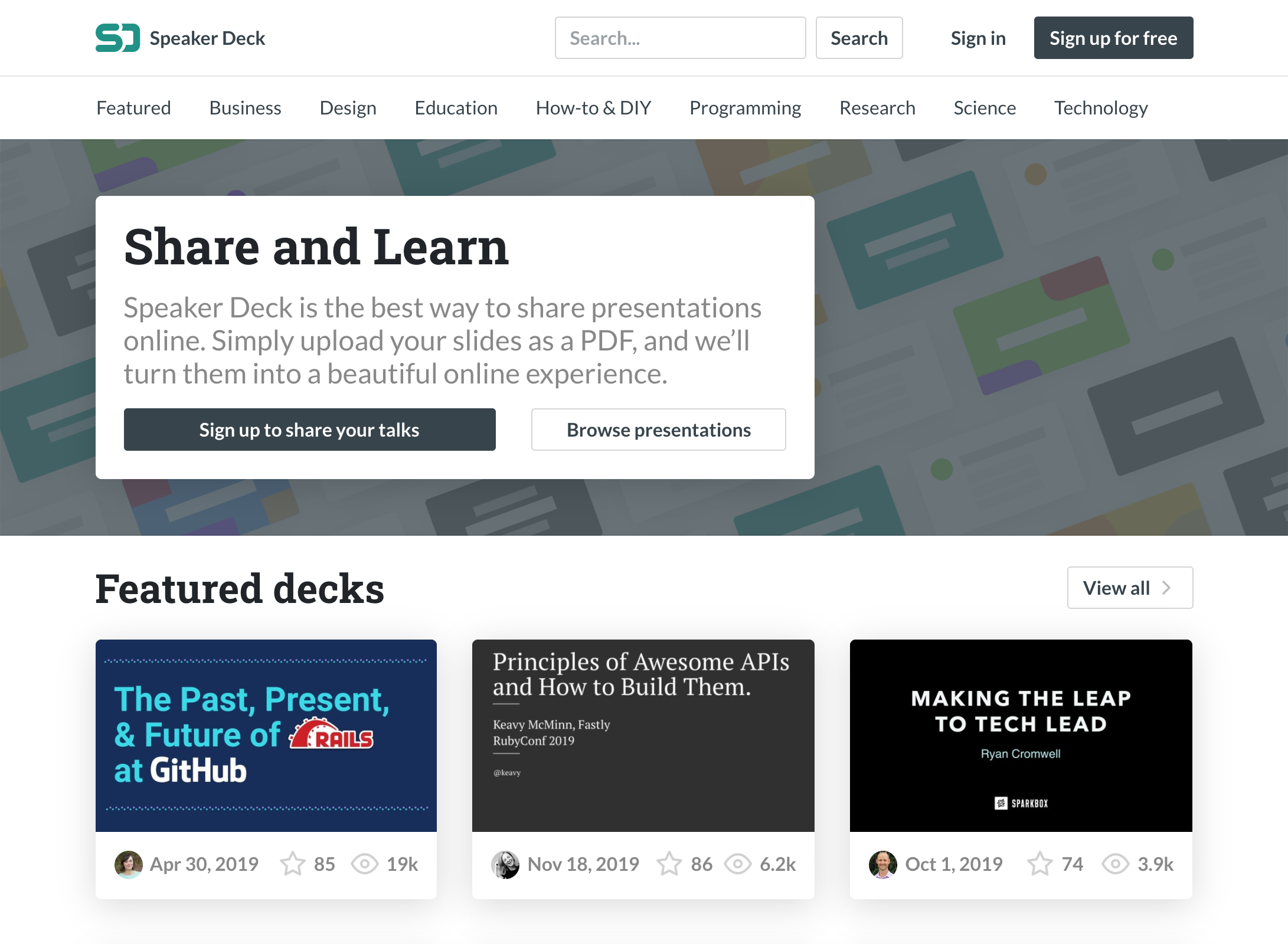The webpage for Speaker Deck prominently features a navigation bar at the top with tabs labeled: **Feature, Business, Design, Education, How-To, DIY, Programming, Research, Science,** and **Technologies**.

In the center of the page is a large rectangle with a blurred background. Overlaid on this is a smaller white rectangle with bold, black text that reads: **Share and Learn. Speaker Deck is the best way to share presentations online. Simply upload your slides as a PDF, and we'll turn them into a beautiful online experience.** Below this text, there are two distinct buttons; the black button is labeled **Sign Up**, and the white button is labeled **Browse Presentations**.

Directly beneath this, in bold black letters, is the heading **Feature Decks**. Below this heading are three rectangular blocks, each highlighting a featured deck:

1. **The Past, Present, and Future at GitHub** – Dated April 30th, 2019.
2. **Principles of Awesome APIs and How to Build Them** – Dated November 18th, 2019.
3. **Making the Leap to Tech Lead** – Dated October 1st, 2019.